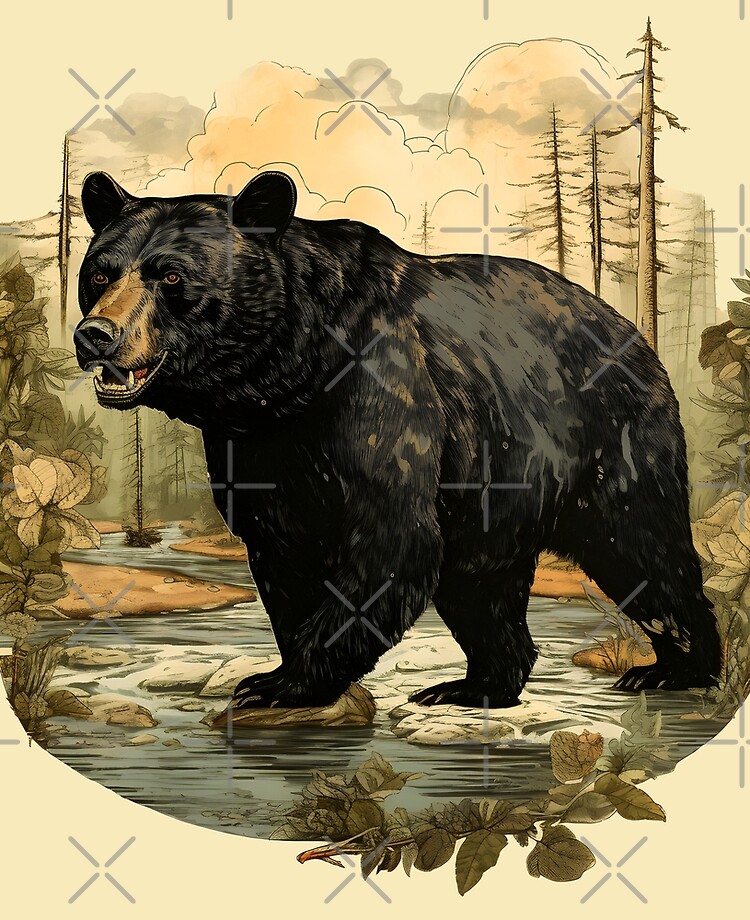The image is a detailed illustration, possibly computer-generated, that depicts a black bear with a brown snout and dark nose making its way across a creek. The bear's mouth is slightly open, revealing its red tongue and white teeth, and it stands with three of its paws on scattered stones, while one paw is immersed in the water, which has a slight blue-gray ripple effect. The background features a natural scene typical of a forested, mountainous area, with large trees stripped of some branches, muted dark green foliage, vines, and decorative flowers. The overall scene is rendered with a vintage feel, with a cream-colored backdrop that enhances the aged aesthetic. Additionally, the entire image is overlaid with numerous X's and plus sign watermarks, likely to prevent unauthorized use, suggesting it might be available for purchase from a website.